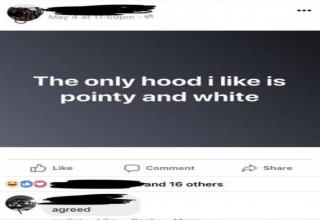The image depicts a social media post overlaid with a dark gray or black banner featuring white text. The username of the individual who made the post is obscured with black lines, likely done using image editing software. The post itself is racially motivated, containing the offensive statement: "The only hood I like is pointy and white." 

Below this post, the usernames of several individuals are similarly redacted with black lines. It indicates that at least 16 users have reacted to the post, as demonstrated by the mention of "some user and 16 others" accompanied by emoji reactions. 

Underneath the original post, another user—whose identity is also concealed with black lines—has commented with the word "agreed," showing support for the offensive message. The small user icon beside this comment is not clear enough to identify the commenter, but it signifies another individual expressing agreement with the racially charged content.